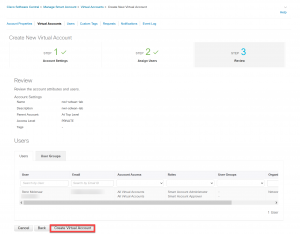The image features a layered user interface on a white background, dominated by various textual and colored elements. In the top left corner, there are multiple lines of gray text—specifically five distinct entries. Below this, another section of gray text appears, followed by a larger block of dark black text consisting of multiple lines: five in the first part, then six, and another two sets of four and five lines of gray text respectively.

In the central area, a segment with a gray background and gray text is visible, which appears to mention "creating an account" or "counting in." This section is partially obscured and difficult to fully decipher. To the right, there's a vertical sequence marked with green numerals one through three. There are checkmarks beside the numbers one and two, which are on a white background, while number three is surrounded by gray.

The left side of the image contains more textual information arranged vertically. This includes six distinct entries of gray text with black accents, although the specific content is unreadable. 

At the bottom of the image, there are clearly visible "Cancel" and "Back" buttons. Adjacent to these is another button with partially legible text mentioning "create an account," framed by a red square. 

Overall, the image displays various sections with text and interactive elements, possibly part of a form or registration interface, though the specific details of the text remain unclear due to visibility and size issues.